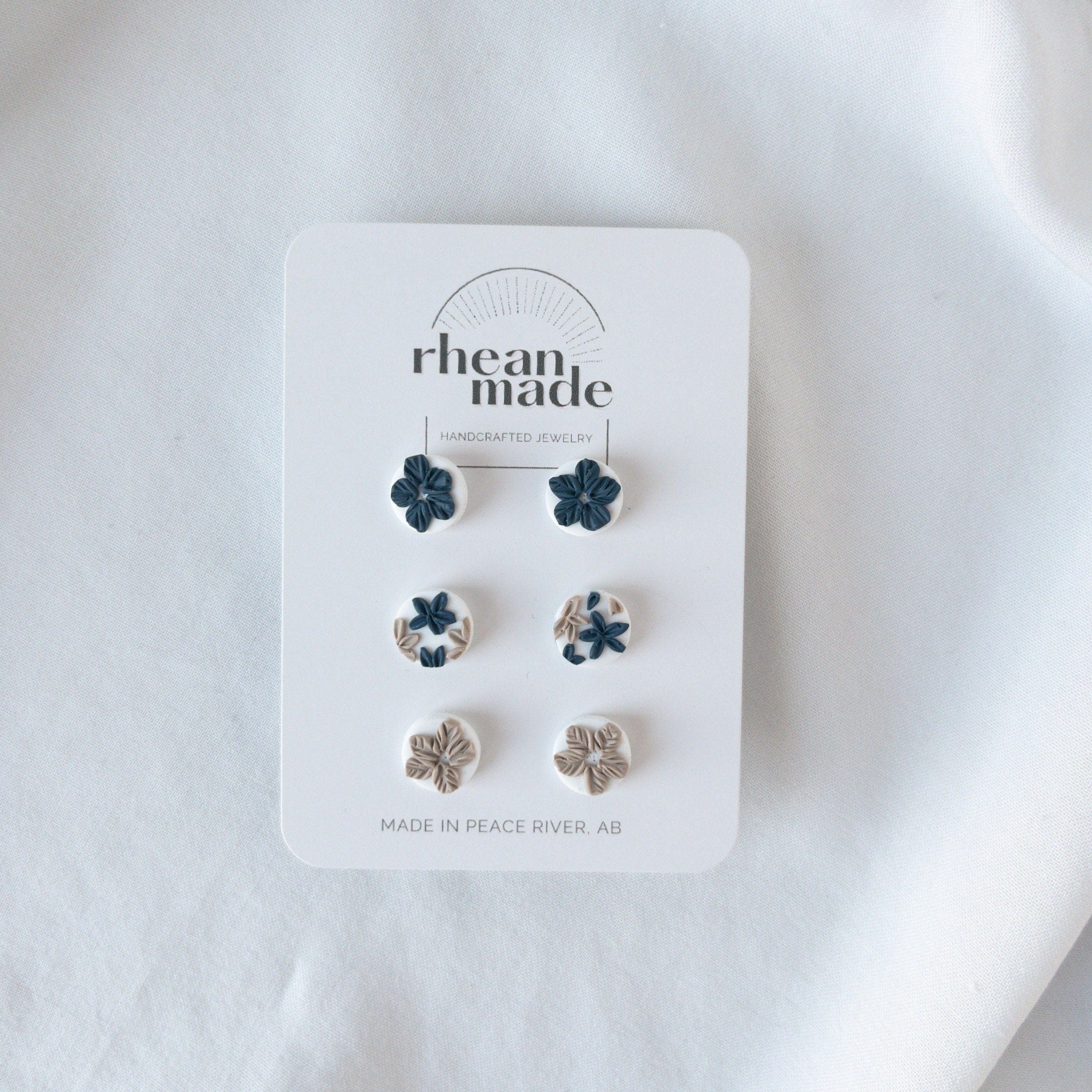This close-up photograph features three pairs of small, handcrafted earrings displayed on a cardboard backing, laid out on a white tablecloth. The card prominently features the brand name "Rhean Made" with a small semi-circle above it, followed closely by "Handcrafted Jewelry." At the bottom of the card, it states "Made in Peace River, AB" in an all-caps, sans-serif font. The top pair of earrings showcases a blue floral design with elements that resemble starfish and coral. The middle pair, matching in design, features brown flower petals instead. The bottom set has circular earrings with a subtle gray floral pattern. This detailed packaging underscores the artisanal quality of the jewelry, highlighting its unique, handcrafted nature.